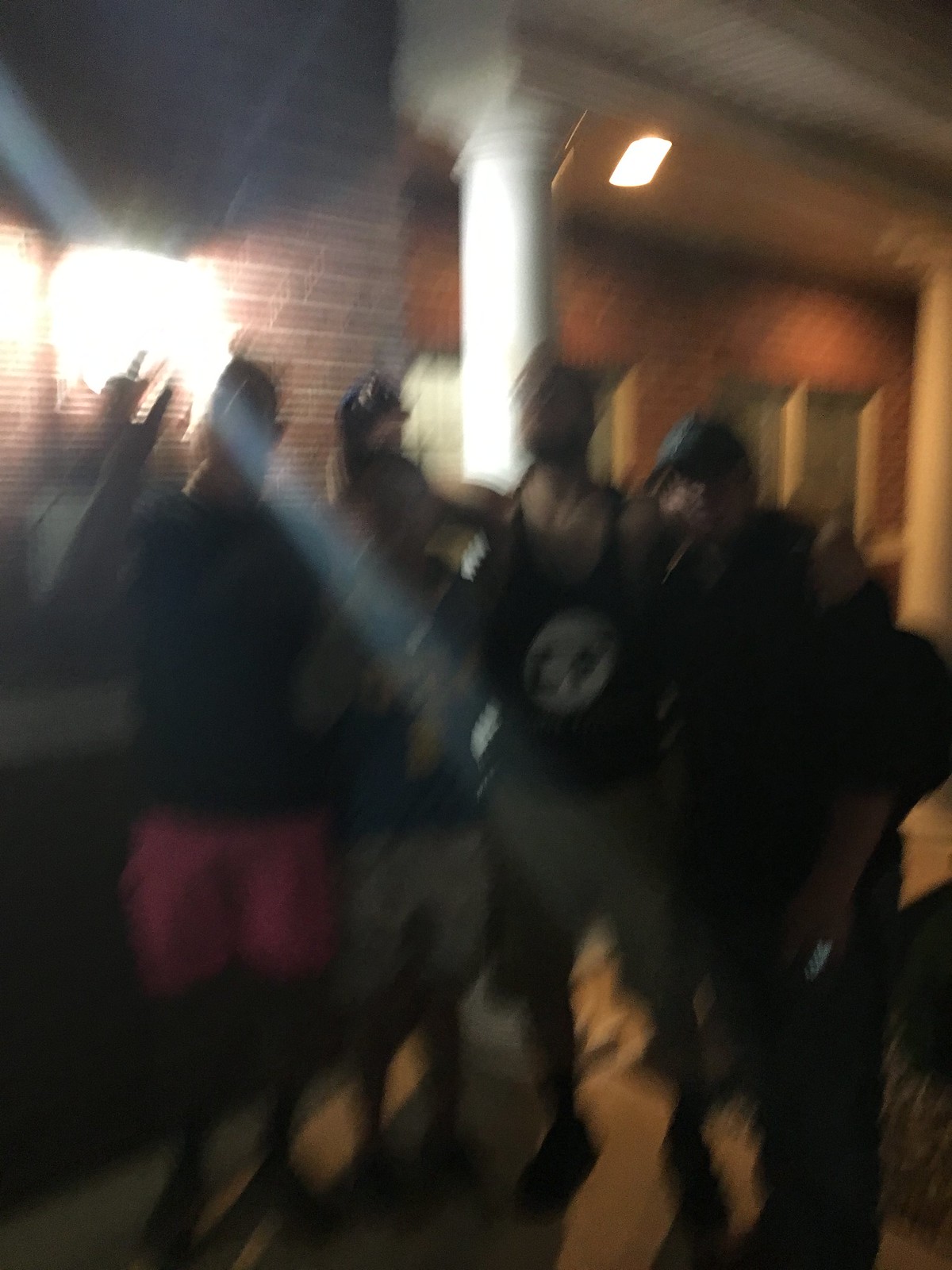A group of four men and a young boy are captured in this dimly lit and slightly blurry photograph. They appear to be enjoying themselves outside a bar or restaurant. The men stand close together in front of a red brick wall with a light fixture mounted above, casting a warm glow on them. The man in the center, notably taller, has his arms around the two men beside him, while the young boy stands in front of him. In the background, additional red brick walls and windows with some illuminated from within are visible, along with a white, round column supporting an overhang. A light from the overhang also contributes to the overall illumination of the scene, highlighting the concrete ground beneath their feet.